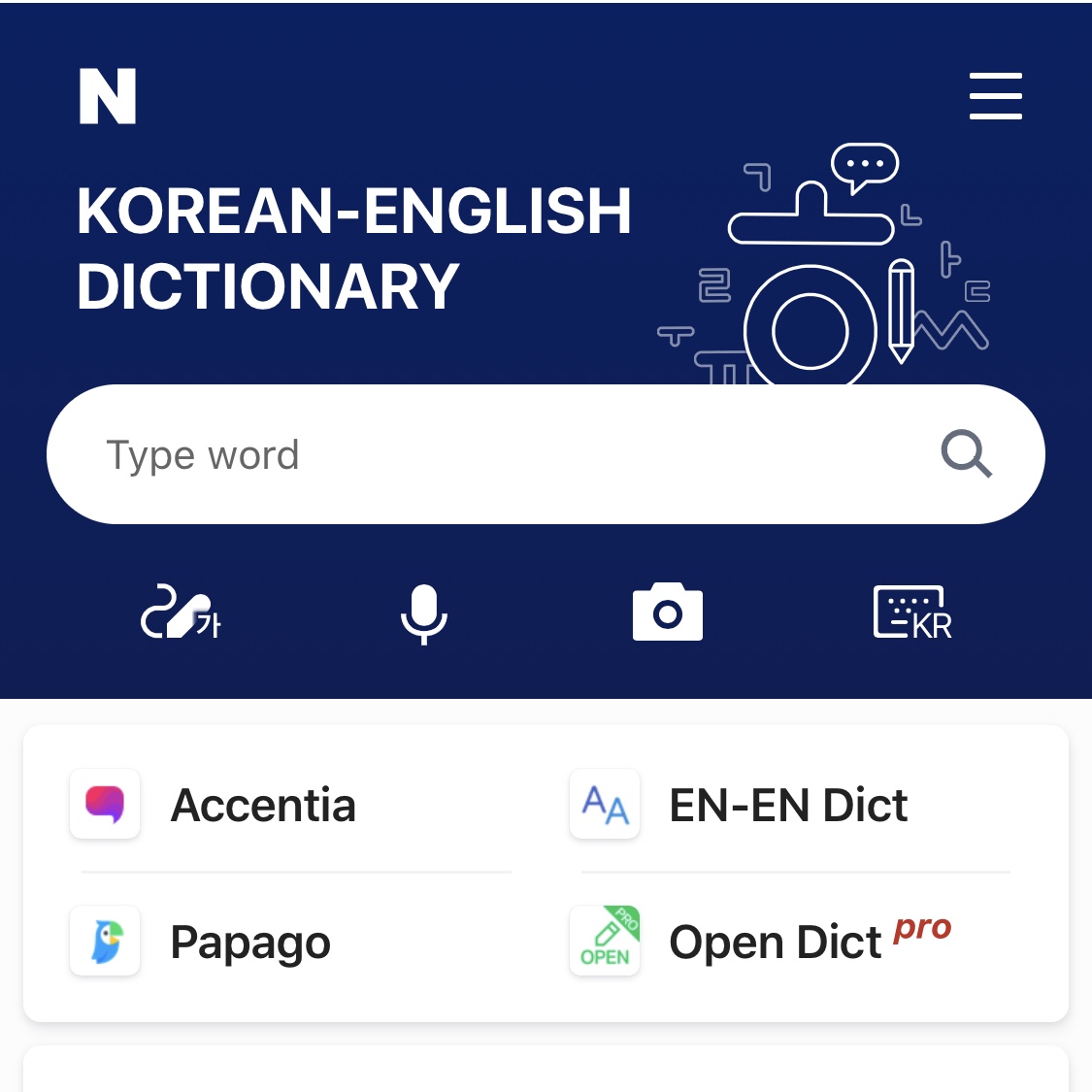The image depicts a user interface with a predominantly white theme interspersed with navy blue and various icons. At the top, a large navy blue square with a thick, capital "N" is present on the left-hand side. Below the "N," the text "Korean-English Dictionary" is prominently displayed in big white capital letters. In the top right corner, there are three small, horizontal white bars indicating the menu.

Adjacent to the text "Korean-English Dictionary," several icons are neatly lined up. These include a white-outlined chat icon with three dots, a circle within a circle, an outline of a pencil, and the outline of a notebook's top. Behind these icons, faintly visible, are random characters like the number "2" and the letter "M."

Beneath this section, a large white banner contains the text "Type word" in gray, alongside a dark gray search icon on the right side. Below this banner, there is an intricate icon depicting a backward "S" with an arrow pointed upwards and two unfamiliar characters, indicative of foreign letters. Accompanying these are additional icons: a white microphone, a camera outlined in white, a box outlined in white with small dots inside it, labeled "KR" in white.

Further down, the interface's bottom part is also white and features the following elements: "Essentia" written in black alongside a white box with a pink chat icon. Below this, the word "Papago" (spelled P-A-P-A-G-O) is accompanied by a white box containing a blue bird with a yellow beak.

In the top right, the letters E-N-E-N-D-I-C-T are displayed next to a white box with two blue "A"s. Under this, the term "Open D-I-C-T" appears, with the word "Pro" highlighted in red. Next to this, a white box with a green outline of a downward-pointing pencil includes the words "Open" in green and "Pro" in white, set against a green background.